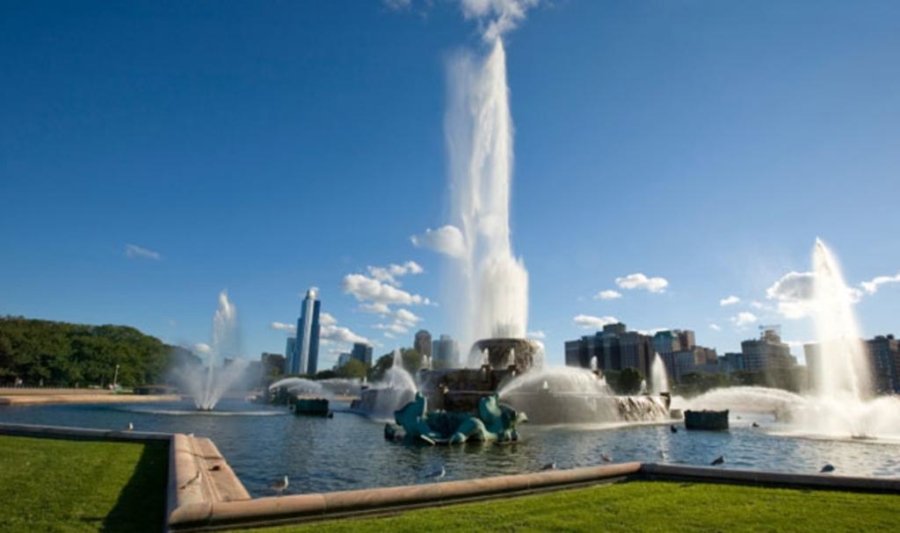This is a color photograph of a large urban fountain complex situated in either a city park or close to a city center. Dominating the foreground, several fountains are visible, with a central one spewing a column of water between 12 and 20 feet high. The fountains are set in a blue pond encased by a gray ledge, which outlines the water area in an intricate pattern starting from the lower left, making several turns as it spans across the image. Grazing the ledge, some gray and white seagulls can be seen, with lush green trees thriving on the left side, indicating a well-maintained park-like setting. The grassy area along the bottom edge of the photo appears freshly mowed, enhancing the vibrant green. Adding to the picturesque scene, green-hued statues, possibly seals or dolphins, also spout water within the fountain ensemble. In the background, tall buildings in tan and gray hues rise against a vast blue sky, which dominates the upper portion of the image. A few fluffy white clouds drift near the horizon, completing the serene urban landscape free of any present people.